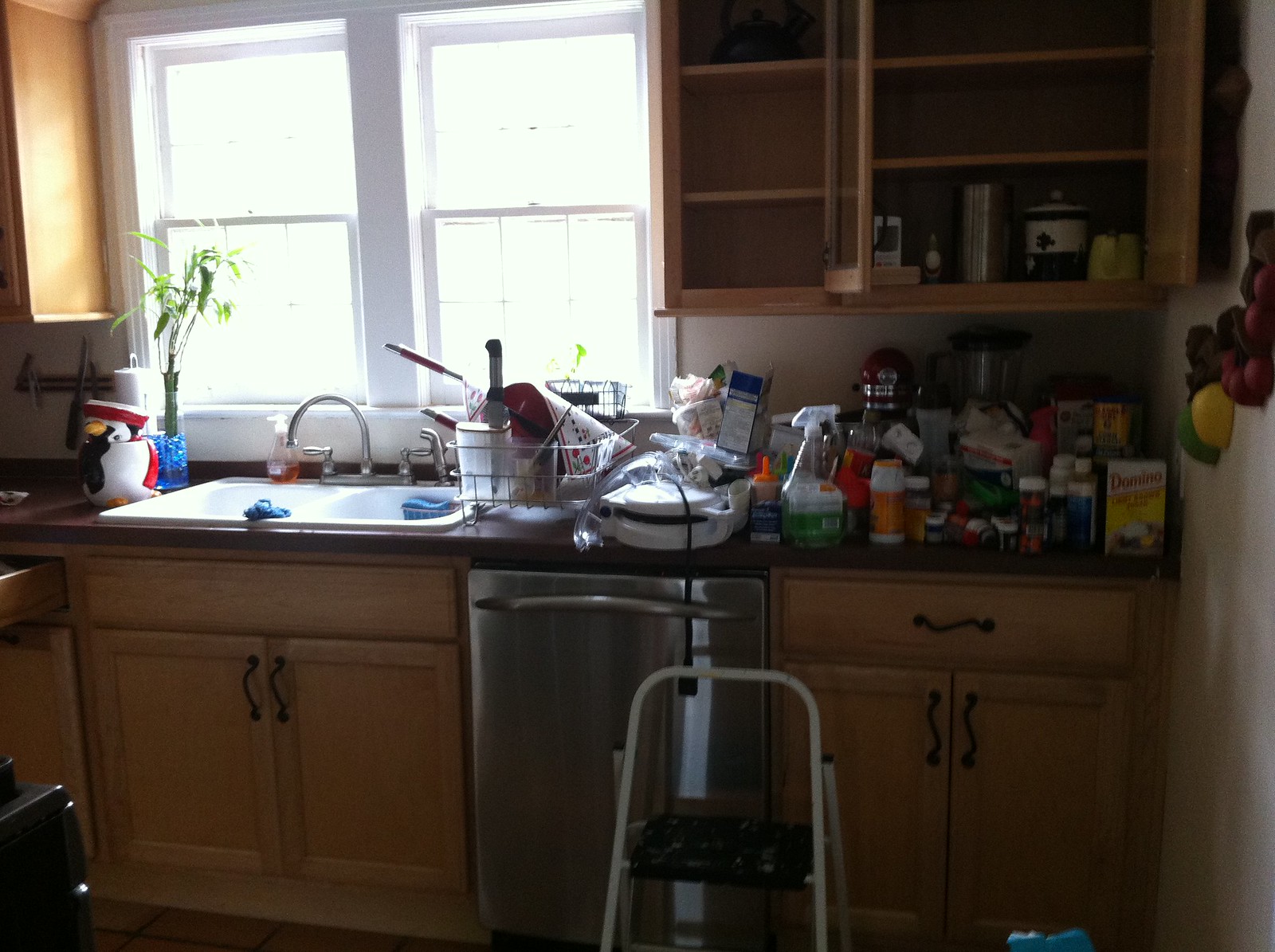The photograph captures a chaotic kitchen scene in the midst of a deep clean. Central to the image is a two-tier step stool, positioned to suggest active use. Above it, the cabinets are mostly empty, except for the bottom shelf on the right. The walls are adorned with whimsical fruit-shaped decorations, adding a touch of charm to the otherwise cluttered space. 

The countertops are crowded with various kitchen items, including a trusty KitchenAid device, a blender, and a spray bottle that faces away from the camera. An upside-down George Foreman grill and a box of Domino brown sugar dominate the scene, surrounded by an assortment of spices, herbs, corn starch, and coffee filters. A drying rack is laden with pots, pans, dishes, and plastic ware, suggesting recent washing activities. 

The cabinets are a light wood color, warmly illuminated by bright sunlight streaming through a window. The sink is conspicuously clear, next to a bamboo plant thriving in a jar filled with marbles and water, and a quaint penguin-shaped cookie jar positioned to the left. Below the George Foreman grill and partially obscured by the step stool is a brushed steel dishwasher, providing a modern touch to the kitchen's rustic appeal.